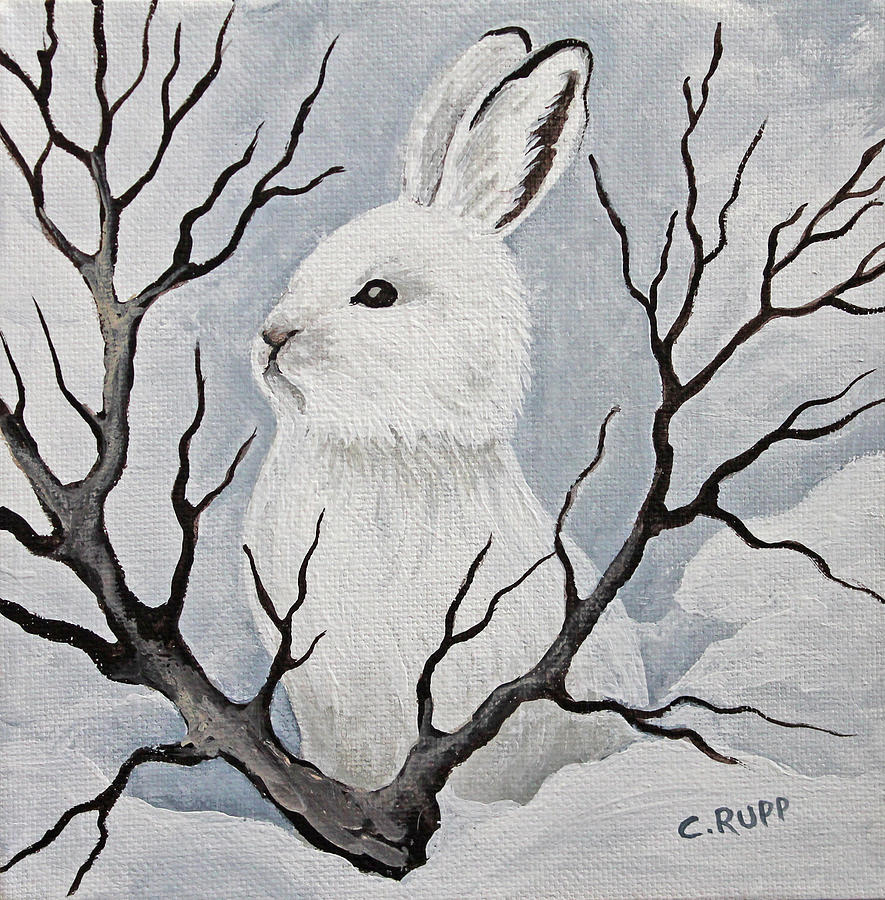The painting, an amateur acrylic work on canvas, captures a small, stylized white rabbit resembling an arctic hare. The rabbit, with its slightly pink nose, prominent black eyes, and a little black lining atop its ears, sits upright in the center of a snowy landscape. A bit of gray shading adds depth to its fur, making it look fluffy and almost pet-like, akin to a magician’s rabbit. The background suggests a cold, wintery scene with a bluish-gray sky. In front of the rabbit extends a barren, leafless brown twig, partially embedded in the deep snow covering the ground. The signature, "C. Rupp," is visible in the bottom right corner of the painting.